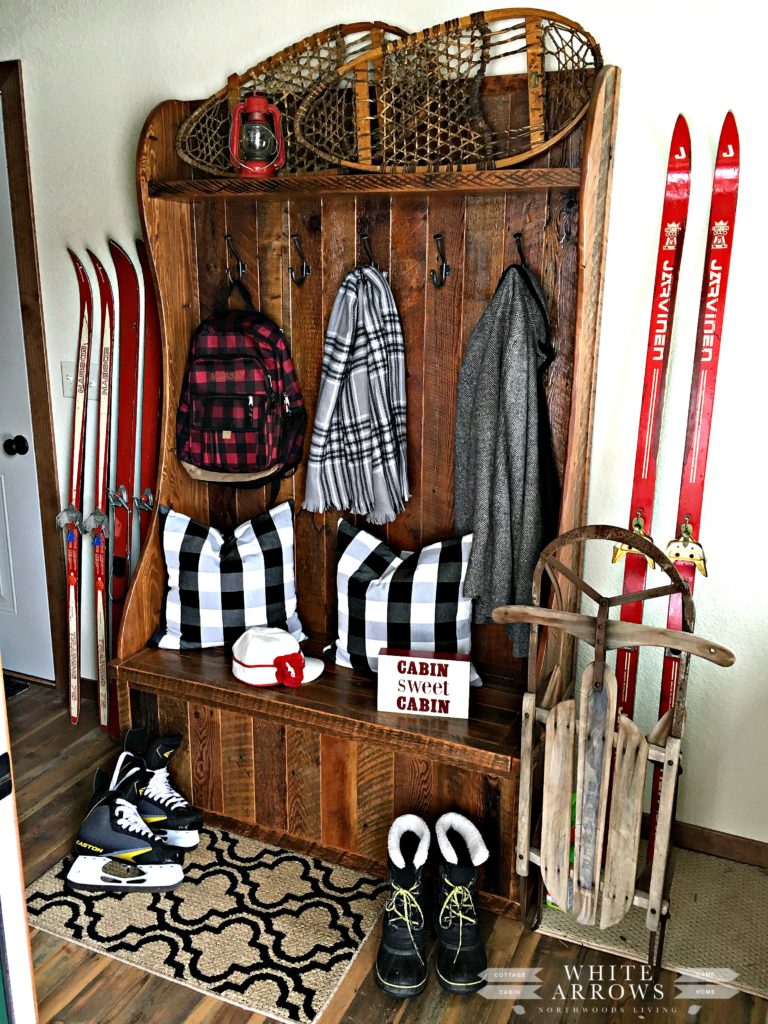This photograph captures a cozy and inviting mudroom or entryway, likely part of a ski lodge or cabin. The space features wooden flooring and white walls, emphasizing a rustic yet clean aesthetic. Dominating the room is a large, possibly handmade wooden bench with a tall back, which serves as a central hub for various accessories and equipment. The bench displays a sign that reads "Cabin Sweet Cabin" and two buffalo black plaid pillows, adding a touch of charm and comfort.

Hanging from the high-backed bench are several items, including a red and black plaid backpack, a checkered scarf, and a lightweight gray jacket, ready for the next outdoor adventure. Above the bench, a shelf holds a small red lantern and some vintage-looking snowshoes, doubling as both decor and functional items.

In the corner to the right, there is an intriguing label that reads "White Arrows," though the rest of the text is unclear. This area is also home to various snow and ski gear: two sets of skis are placed against the wall, another pair of taller skis stand nearby, and between them sits an old-fashioned sled. Completing the winter-ready setup are a pair of black-lined snow boots and black ice skates laid out on a rug.

A white door is situated to the left of the scene, with a light switch partially obscured by the propped-up skis. The overall composition reflects a warm and well-organized space, designed to cater to snowy escapades with ease and style.